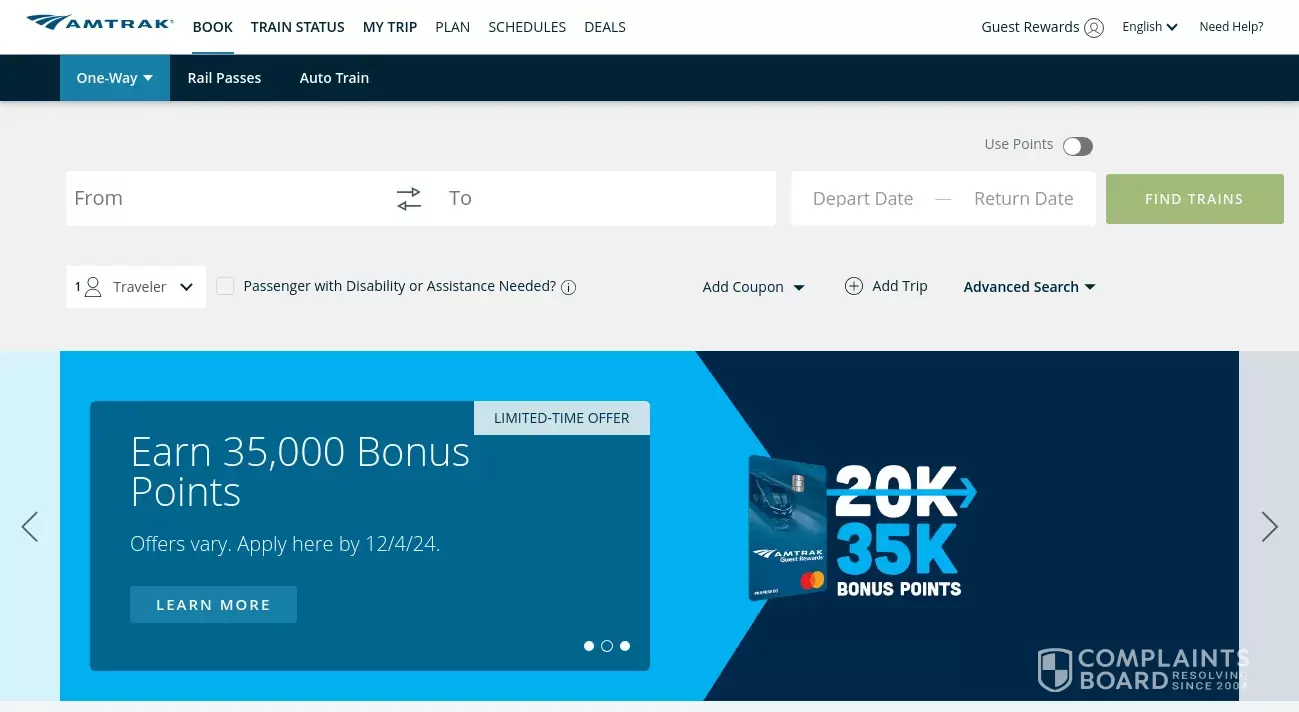**Detailed Caption for Amtrak Website Screenshot**

The image displays a screenshot of the Amtrak website. At the top of the big square picture, there is a long, thin blue bar that gets darker towards the right. In the upper left corner, the Amtrak logo is prominently featured with "AMTRAK" written in white, all-caps text. Directly to the right, white text spells out "JOIN," followed by a white bar labeled "SIGN IN." Adjacent to this, a dropdown menu offers language selection, and another white box with blue letters reads, "Need help? Ask Julie," accompanied by a microphone icon and a magnifying glass on the far right.

Below this section, another menu embedded in a long blue bar lists several options in white, all-caps text: "DESTINATIONS," "EXPERIENCE," "DEALS," "SCHEDULES," and "GUEST REWARDS." On the far right of this menu, icons for CLOCK and TRAIN STATUS, along with a pencil icon labeled "MY TRIP," are also visible.

Directly below, the user is presented with a black line featuring three selection options. The first option, highlighted in blue with white text, is "ONE WAY," while the other two options are "RAIL PASSES" and "AUTO TRAIN."

The main body of the site has a gray background. A white bar in the top left corner indicates input fields "FROM" and "TO," featuring black letters and two arrows facing opposite directions. To the right, white boxes are provided for "DEPARTURE DATE" and "RETURN DATE," including a toggle for using points. Beside these, a grayed-out green box that reads "FIND TRAINS" suggests it’s currently unclickable, flanked by a person icon indicating one traveler, and subsequent clickable options for adding travelers, specifying passenger needs, or conducting an advanced search.

Dominating the center of the image is a rectangular photo of a Caucasian woman with shoulder-length brown hair, seated and gazing out a train window at a cityscape. Her reflection appears in the window, which is superimposed with a transparent blue box. The text on this box reads, "ELEVATE YOUR TRAVEL EXPERIENCE. Place a bid to upgrade your reservation to a premium class of service." Below, a blue box with white, all-caps letters states "LEARN MORE," featuring three small circles indicating navigation slivers, with sideways-facing V's for additional navigation on either side.

Below the central image, three additional pictures are arrayed:
1. The first image on the left is an aerial shot of a nature escape during fall, faintly showing a train. The Amtrak logo in the bottom right corner promotes the "Amtrak Gift Card" in a blue box. Subtext encourages gifting Amtrak travel, emphasizing that the cards are easy to redeem and never expire, with a "PURCHASE NOW" link in blue.
2. The middle image is a sunset view over flat-country train tracks, headlining "SAY HELLO" in large white letters and "200,000 BONUS POINTS" below. It promotes earning up to 200,000 bonus points with the Amtrak Guest Rewards Preferred Mastercard, accompanied by a credit card image and additional text encouraging users to learn more.
3. The third image portrays an African-American family of three inside what seems to be a train station or suite. It advertises "FIRST-CLASS PRIVATE ROOMS" available on many routes across the country, with a "LEARN MORE" link in blue below the description.

On the far right of the image, a scrollbar indicates the page is at the top. In the far lower left, the word "FEEDBACK" appears on a vertically-oriented blue bar, encouraging user input.

This detailed layout encapsulates the design and content of the Amtrak website’s main page, providing a comprehensive visual and textual overview.